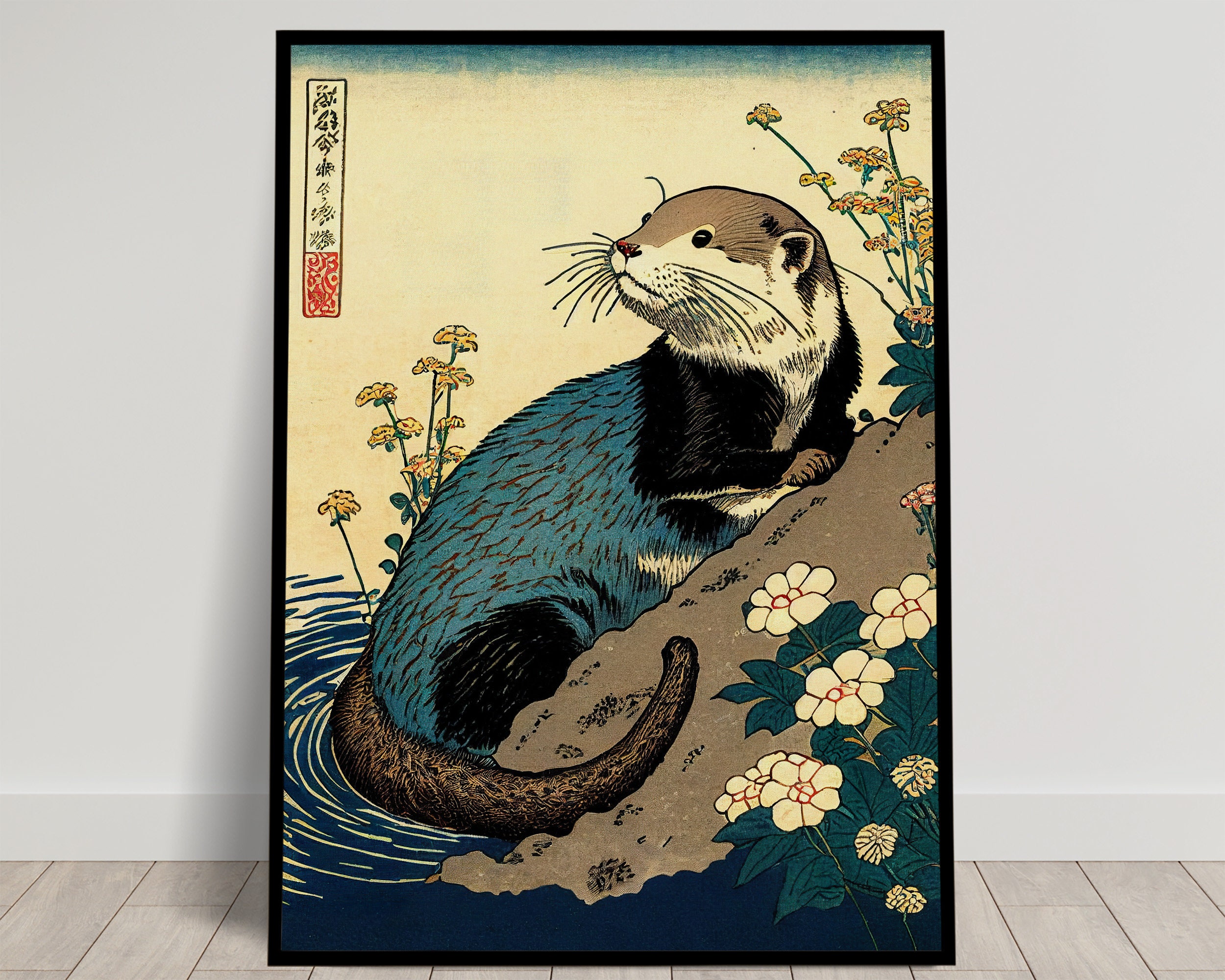The image depicts a staged indoor scene with a wooden plank floor and an off-white wall illuminated by artificial light. Leaning against the wall is a large rectangular painting almost human height and about three to four times as wide, featuring a scene by the water's edge. The painting, set in a black frame, portrays a large, whiskered rodent-like creature, possibly an otter or muskrat, climbing out of the water onto a sloping bank covered in yellow and white flowers. The creature has a distinct coloration: a light brown upper body, a white patch on its lower head and neck, dark brown shoulders and arms, blue torso, brown paws, black hind legs, and a grayish tail. It gazes to the left with beady black eyes. In the upper left corner of the painting, there's writing in an Asian language, presumably Japanese or Chinese, alongside a red rectangle. The setting, with its intentional composition and color contrast, suggests a carefully considered artistic arrangement.